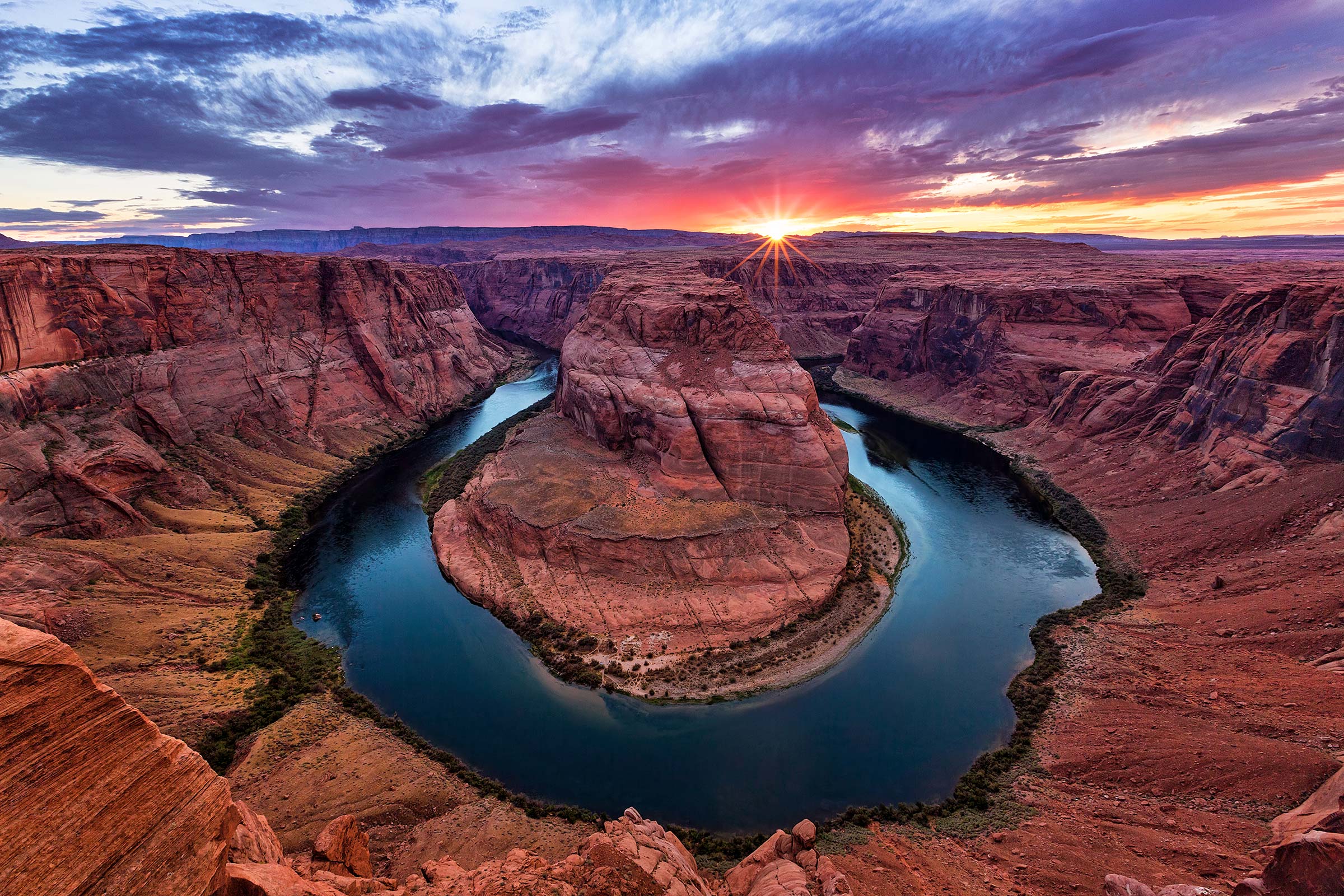This professional photograph, taken from a high vantage point, captures a stunning, canyon-like landscape during either sunrise or sunset. Dominating the scene are a series of mountainous, reddish brown and orange stone formations, including a prominent central mountain surrounded by a U-shaped body of crystal-clear, blue water that appears like a natural moat. The rocky terrain is predominantly bare, with sparse green vegetation and shrubs clinging to the water's edge. The horizon reveals an endless expanse of similar rugged, hard granite cliffs. High above, the sky dazzles with a spectrum of colors – gray, purple, pink, orange, red, yellow, and gold – as the sun, a diminutive golden star, emits radiant beams in multiple directions, creating a magical ambiance that blends with the vivid cloudscape.